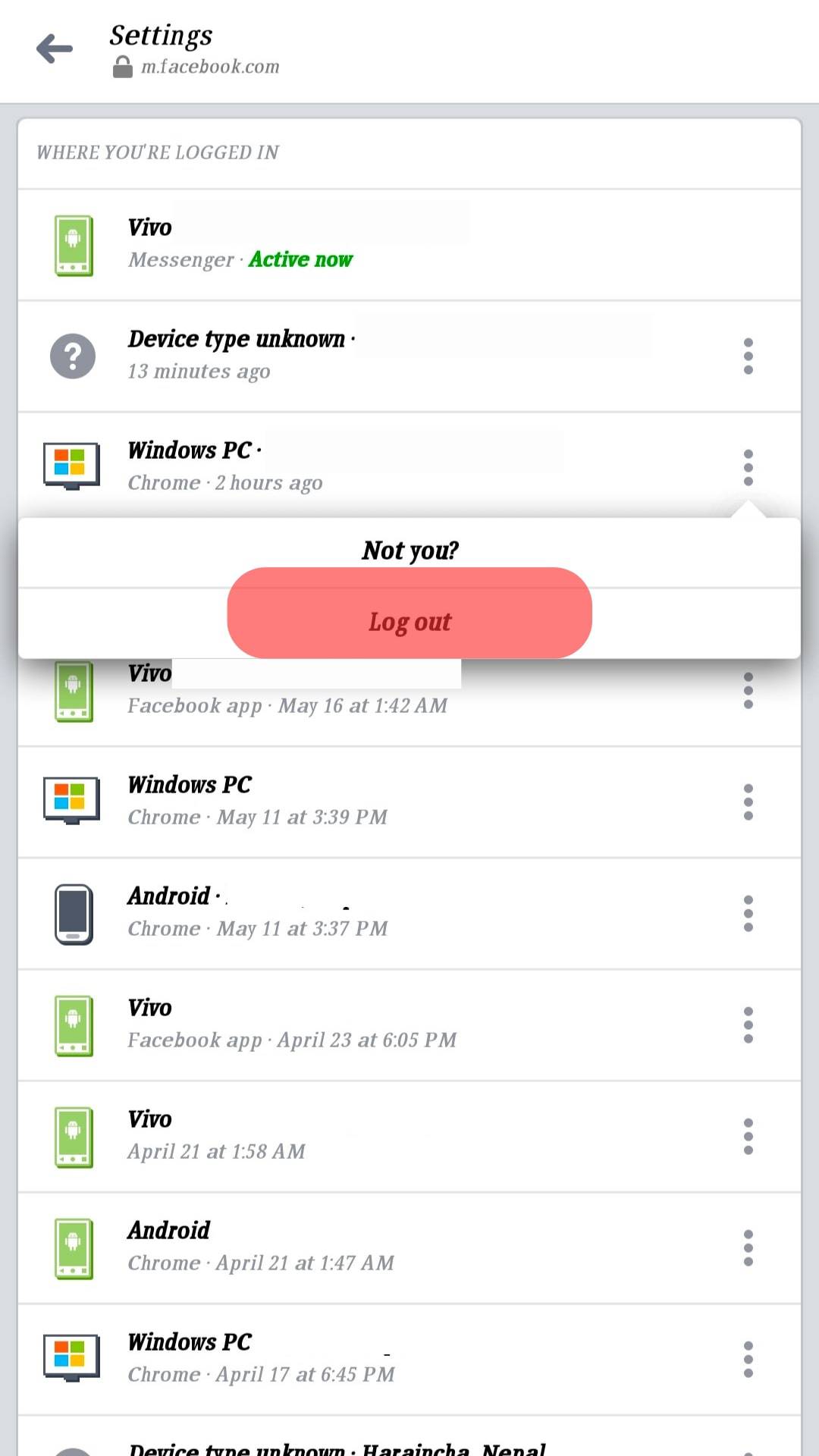The image displays the settings interface of a Facebook account accessed through a web browser. In the upper left corner, the word "Settings" is shown in black font, with a lock icon and the URL m.facebook.com in smaller, gray text below it. The central part of the image features a white background box containing a vertical list of ten items, each representing different devices or sessions where the user is logged in. This list is labeled "Where You're Logged In."

A prominent white pop-up box is pointing towards the third entry in the list, labeled "Windows PC." Underneath this label, it indicates that the session was active on Chrome two hours ago. The pop-up box specifically targets the three vertical dots located on the right side of this bar. The content of the pop-up includes the text "Not you?" followed by a question mark, and an option to "Log Out," highlighted within a red bubble.